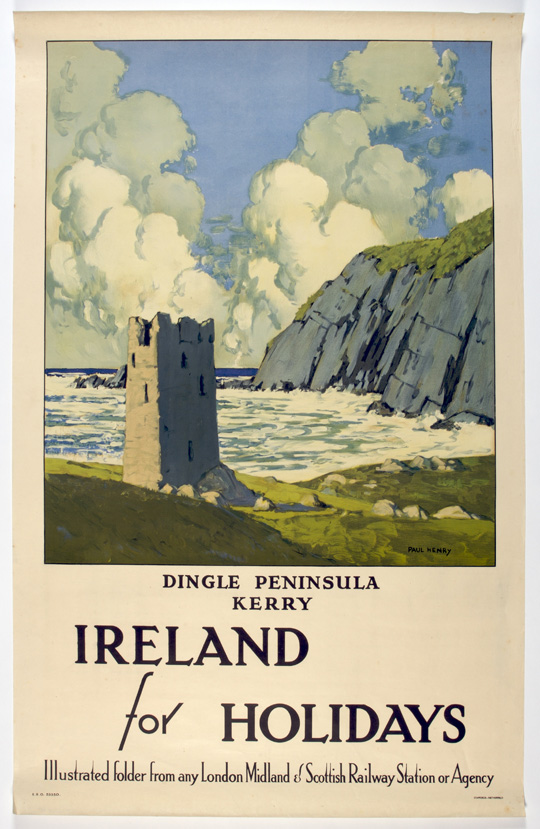This vintage-style poster of Ireland presents a striking hand-drawn scene featuring the Dingle Peninsula in Kerry. Dominating the foreground is a weathered, ancient tower, evocatively set against green low hills dotted with rocks. The ocean, appearing turbulent with foamy waves, crashes against distant gray cliffs that boast verdant grassy tops. The sky above transitions from a light blue hue to a darker cobalt blue at the horizon, adorned with fluffy, billowy clouds. Signed by the artist, possibly with the last name Henry, in the lower right corner, the poster prominently displays the text: "Dingle Peninsula, Kerry" in black capital letters. Below, in larger lettering, it enthusiastically declares "Ireland for Holidays." The bottom section reads, in smaller text, "Illustrated folder from any London Midland and Scottish Railway Station or agency." The overall poster is set against a tannish background, suggesting it might originally be the cover of a pamphlet or brochure for the railway.